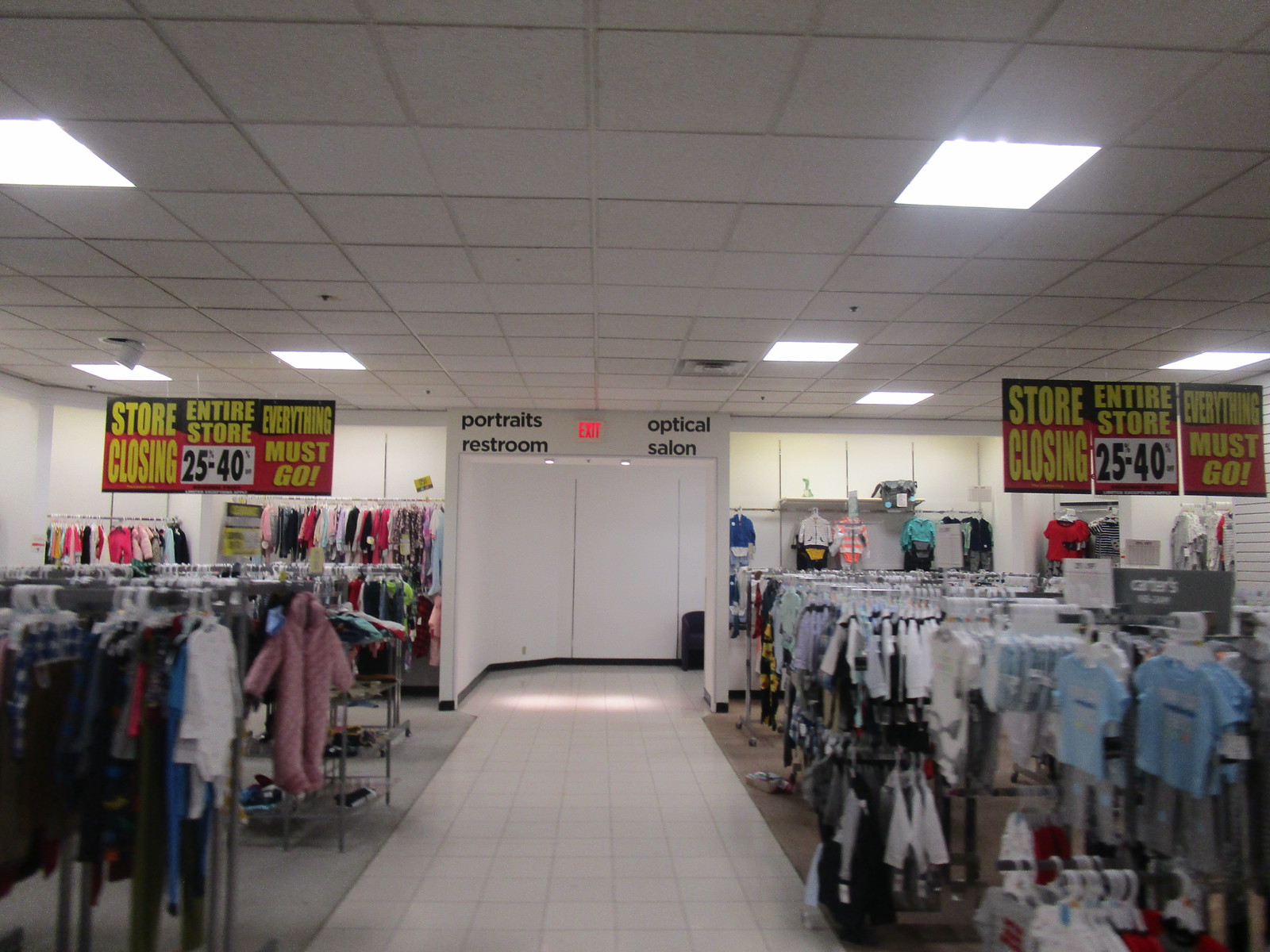In this photograph captured from the central walkway of a department store's clothing section, the viewer's gaze is directed straight ahead. The image showcases the store's various departments and well-arranged displays. The path taken by shoppers is flanked on both sides by carpeted flooring, adorned with meticulously organized displays featuring an assortment of small-sized clothing items. A clear sign is visible in the middle distance, suspended above a doorway. On the left side of the sign, it reads "Portraits Restroom," directing customers towards the facilities. On the right side of the sign, it indicates the "Optical and Salon" section of the store, guiding visitors to additional services. The overall scene exudes a sense of order and accessibility, highlighting the store's commitment to providing a comprehensive shopping experience.